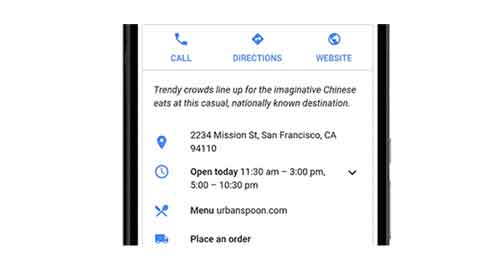Here is the cleaned up and detailed caption for the screenshot image:

---

The image captures a compact screenshot from a map application displaying a restaurant site. The screenshot is a small square framed by moderately thin black banners on both the right and left edges. Within the black banner at the top, there is a thin gray rectangular area housing three distinct icons: 

1. On the left, a phone icon labeled "call."
2. In the center, an icon with an arrow labeled "directions."
3. On the right, a globe icon labeled "website."

Beneath this, enclosed in another thin gray rectangle, the text reads: "Trendy crowd line up for imaginative Chinese eats at this casual nationally known destination." 

Following this description, there is a series of information icons and details:
- A blue location marker icon appears to the left of the restaurant's address in San Francisco, California.
- A clock icon indicates the restaurant's operating hours, stating "Open today."
- Below, a crossed knife and spoon icon accompanies the text "Menu" linking to urbanspoon.com.
- Lastly, a truck icon prompts users to "Place an order."

---

This caption provides a structured and detailed interpretation of the visual elements within the screenshot.